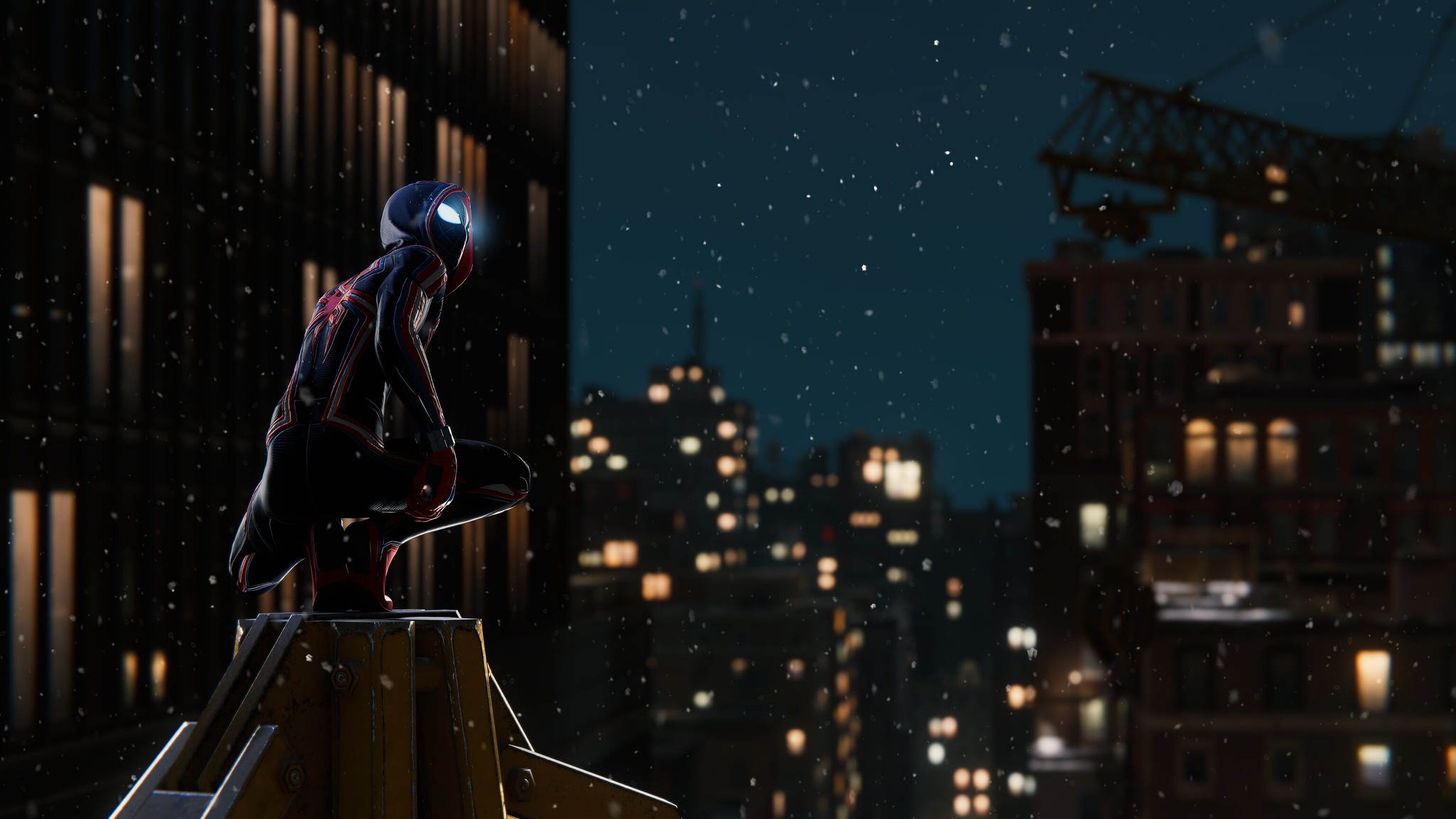In this striking nighttime cityscape photo, towering skyscrapers stand illuminated against the dark sky, with their windows aglow in warm white and yellow lights. To the right, a construction crane looms, adding an industrial element to the urban scene. In the foreground on the left, a concrete pedestal rises prominently, providing a perch for a mysterious figure. This individual, clad in a skin-tight suit complete with a hood, crouches on their knees. Their eyes emit an eerie, bluish glow, lending an otherworldly air to their presence. A distinctive red mark adorns their back, hinting at a unique identity or purpose. The figure's gaze is focused intently to the right, directed at an unseen point just outside the frame of the photograph, creating an intriguing sense of anticipation and storytelling.